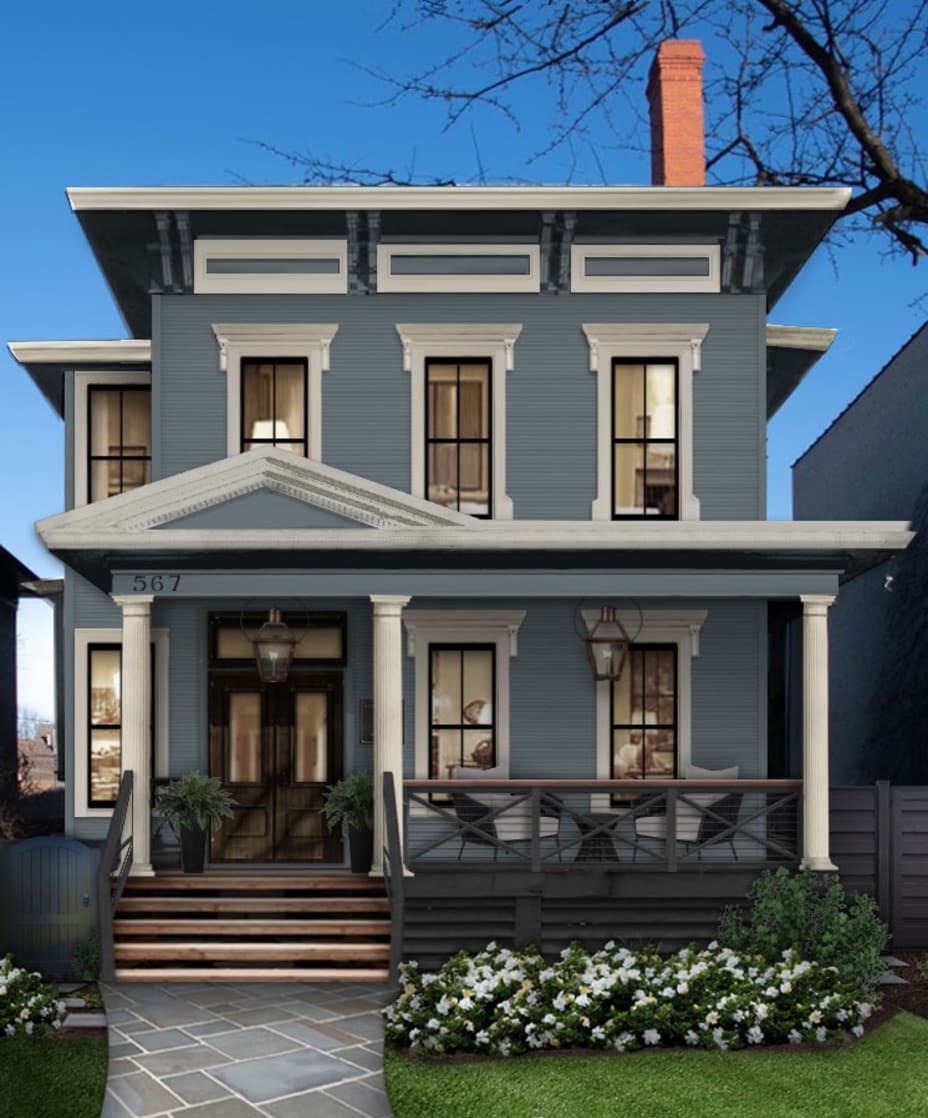This color photograph captures the front view of a beautiful, two-story saltbox-arts-and-crafts style home. The exterior of the house is a muted blue or gray color, accentuated by a white trim around the windows and roof gutters. The house features a meticulously landscaped front lawn with green grass and a small flower bed filled with white flowers on the right side. A paved walkway leads up to the front porch, which is supported by three white-painted columns. 

The porch houses two chairs next to a small table, positioned in front of two white-framed windows. Wooden steps, flanked by two potted ferns and a small black gate on the left, lead up to a black front door with the house number "567" displayed in black on the upper left part of the stairs. Above the porch are three additional windows, also framed in white, with matching white eaves. A brick chimney can be seen extending from the roof, complementing the home's classic yet inviting facade. The scene is set against a beautifully clear blue day, enhancing the home's welcoming and well-maintained appearance.